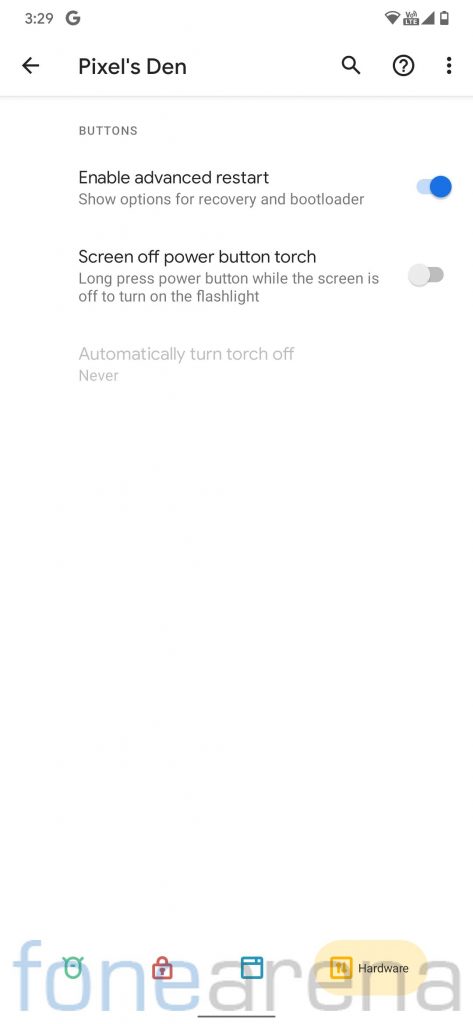Here's the cleaned-up, detailed caption for the image:

The screenshot displays the settings section of an application on a smartphone. The background is white, and the time is shown at 3:29 PM at the top of the screen. The Google logo is visible in the top left corner, while icons representing Wi-Fi, cellular signal, LTE, and battery level are aligned on the top right.

Below this, a back arrow is located on the left side, and the text "Pixels Din" is written in black. On the right side, there are three icons: a search icon, a help (question mark) icon, and a list (menu) icon.

Further down, there are several toggle buttons. The "Enable Advanced Restart" button is highlighted in blue, indicating that it is turned on. Below that, there are options for "Search or Screen Off," "Power Button," and "Torch," which are currently turned off. Additionally, the setting for "Automatically Turn Torch Off" is set to "Never." At the bottom of the screen, the text "Phone Our Arena" is displayed.